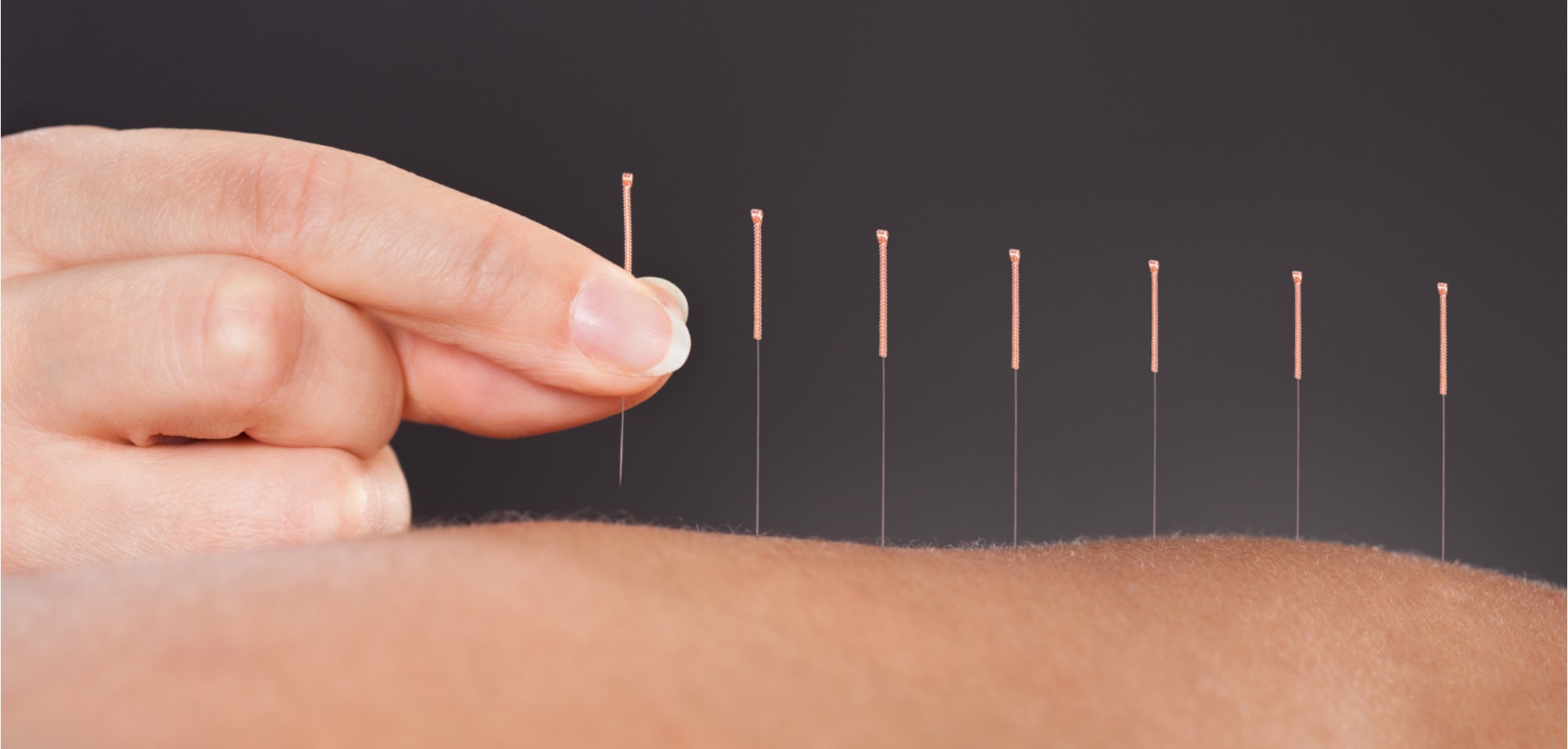A close-up image shows a Caucasian arm with a slightly grayish hue and small white hairs. Seven thin acupuncture needles with yellow tops are inserted into the skin, beginning slightly left of center and extending to the right. On the left side of the image, two fingers, potentially female based on their long and clean nails, hold another needle poised just above the skin, ready for insertion. The background is a solid medium gray, providing a stark contrast to the detailed texture of the arm and the delicate needles.